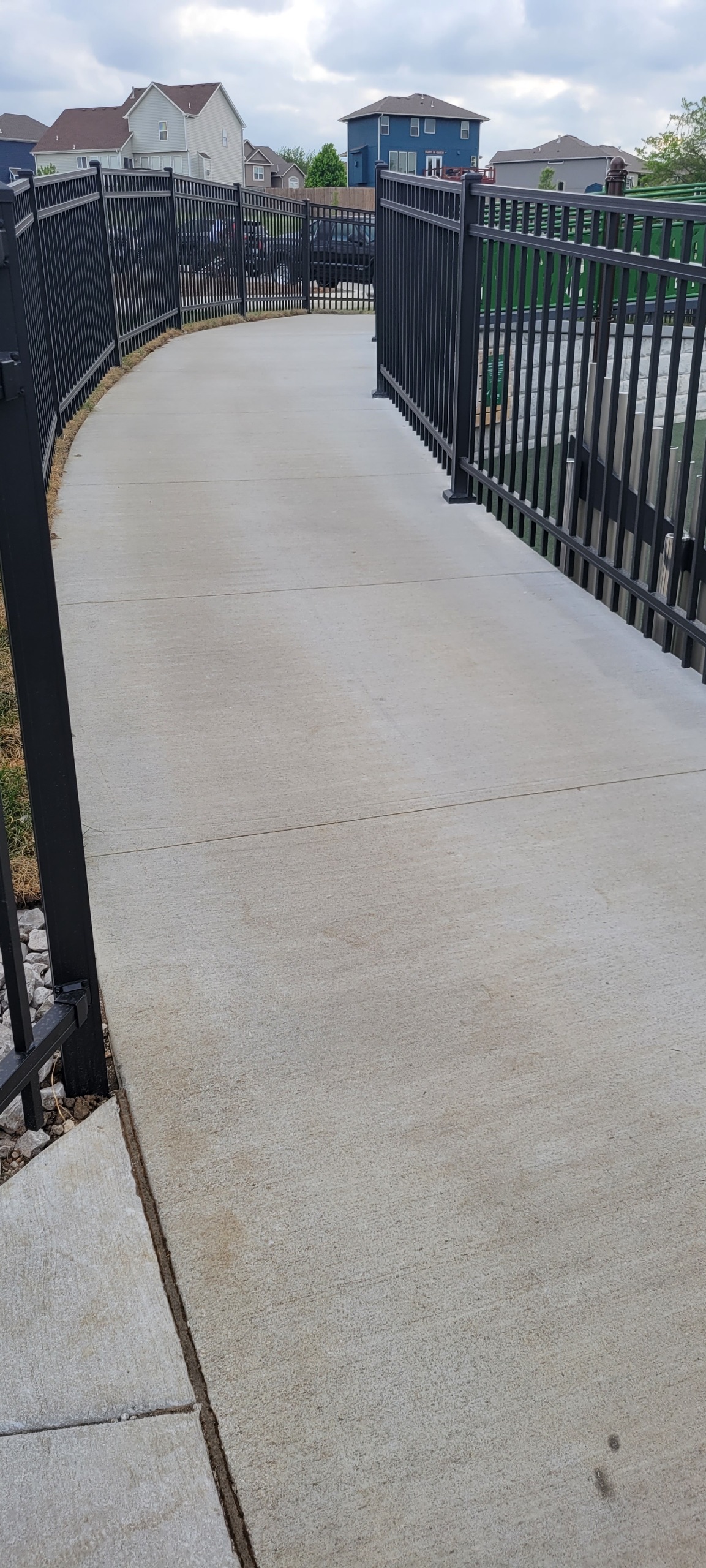This photograph captures a narrow concrete sidewalk flanked by black wrought iron fencing on either side. The perspective shows the sidewalk curving to the right, giving the appearance of depth and an inviting path ahead. The fenced walkway hints at an elevated structure, possibly an overpass or bike path, and adds a sense of safety. Surrounding the path, patches of grass suggest the season might be fall or winter, indicated by its browning hue. In the background, a series of typical suburban two-story houses of varied colors, including brown and blue, are visible under a gray, overcast sky. The scene is devoid of any people or animals, instead focusing on the tranquil suburban setting. Additionally, there is a hint of a retaining wall or possible stairs through the fence, enhancing the layered composition of the neighborhood. This detailed, vertical composition offers a glimpse into a quiet suburban area, potentially near a resort or country club, as indicated by a blue building with a sign in the far background.